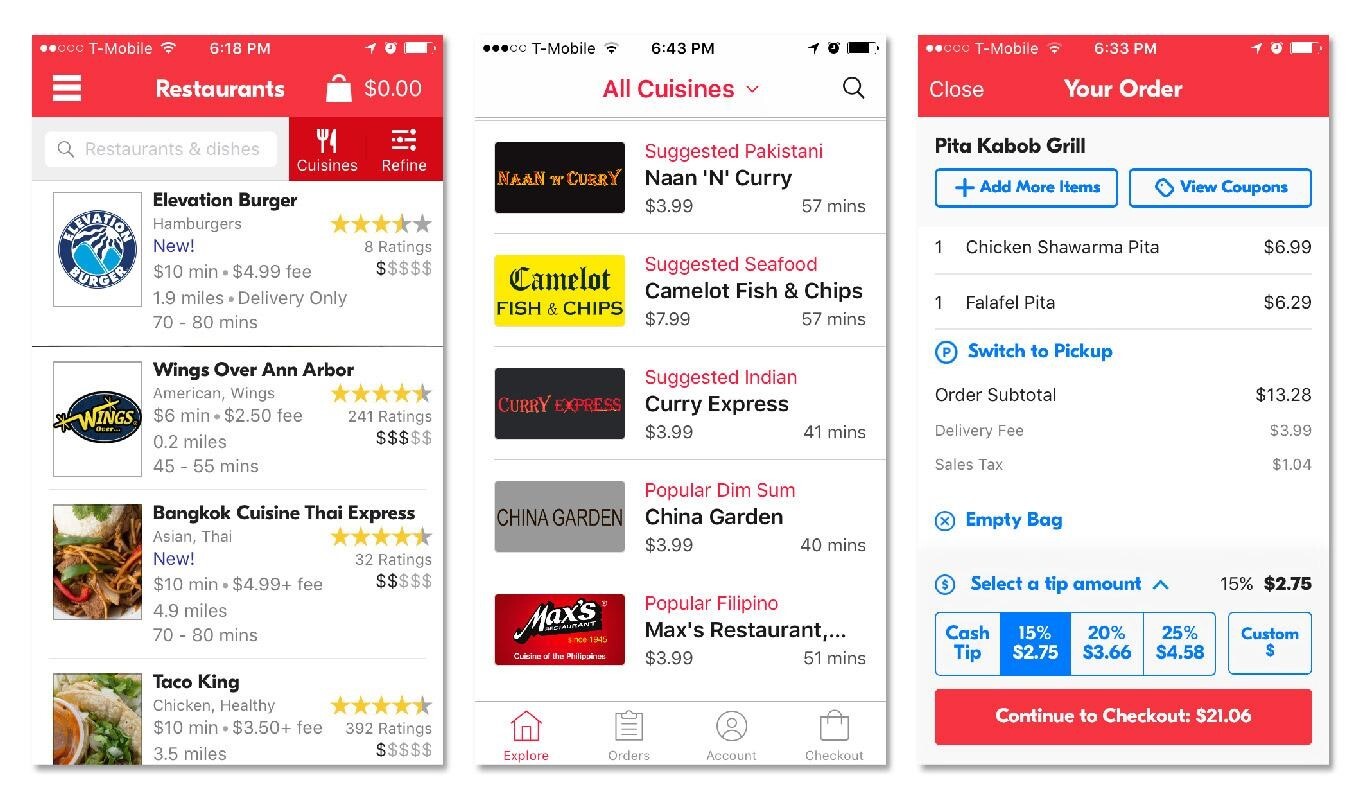The image displays multiple webpages, each providing different types of information. On the left-hand side, a webpage showcases a search for restaurants under the heading "T-Mobile" with the timestamp of 6:18 PM. This page is formatted as a rectangle and lists various cuisines and eateries. "Elevation Burger" features hamburgers, "Wings Over Ann Arbor" offers American wings, "Bangkok Cuisine Thai Express" serves Asian and Thai dishes, and "Taco King" provides chicken and healthy options.

The central section of the image features another rectangular webpage, predominantly white, with a search box labeled "All Cuisines" in pink lettering. This page lists different cuisines and restaurant suggestions: "Pakistani" cuisine is represented by "Naan and Curry," "Seafood" by "Camelot Fish and Chips," "Indian" by "Curry Express," "Dim Sum" by "China Garden," and Filipino" by "Max's Restaurant."

On the right-hand side, there is a third rectangular webpage, also predominantly white but with a red header stating "Close" and "Your Order." This page details an order for "Pita Kebab Grill" including a Chicken Shawarma Pita priced at $6.99 and a Falafel Pita at $6.29, bringing the order subtotal to $13.28. Additional charges include a delivery fee of $3.99, a sales tax of $1.04, and a 15% tip amounting to $2.75. At the bottom of this webpage, a red button allows the user to "Continue to Checkout" with the total amount calculated at $21.06.